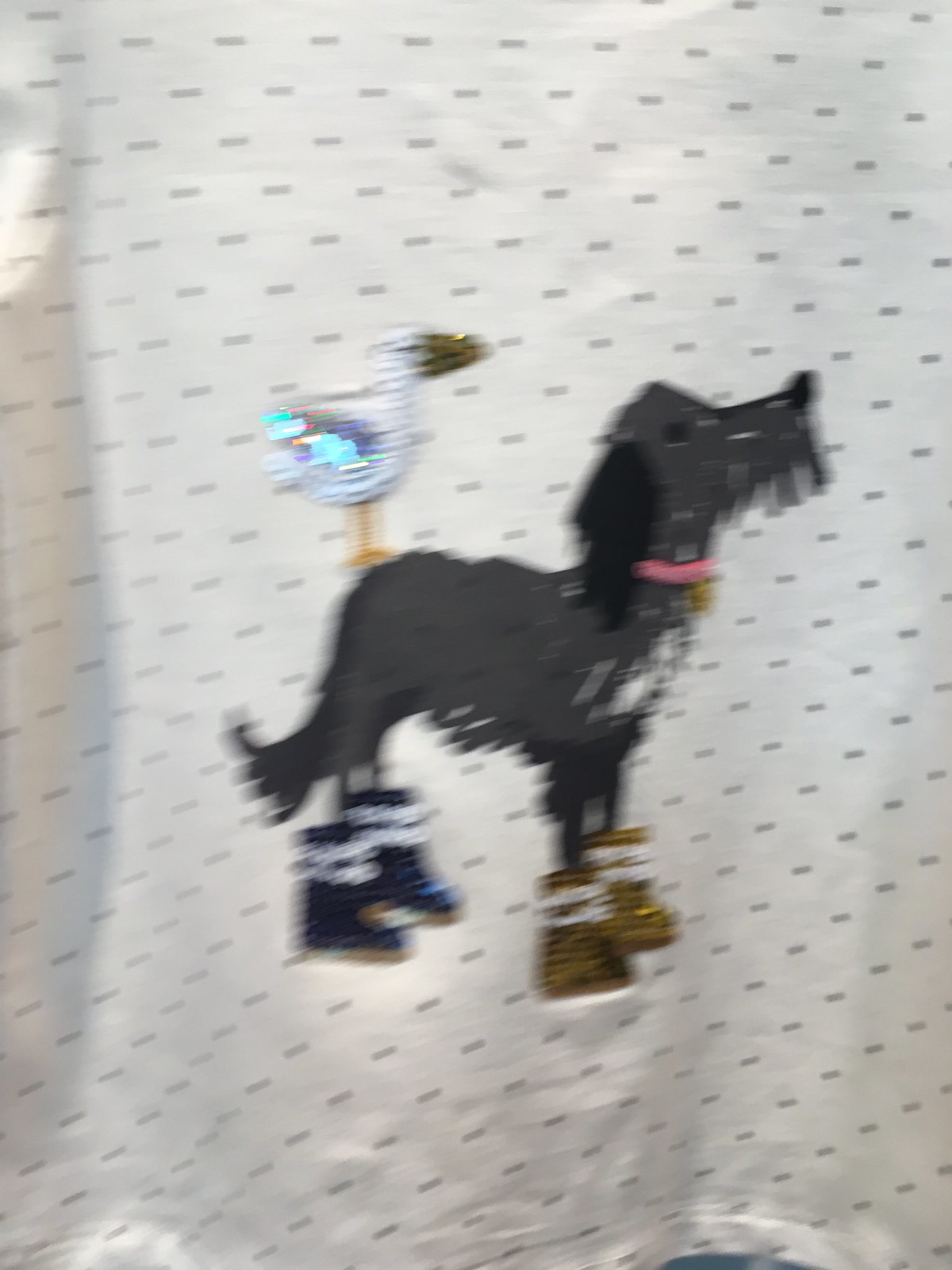This image captures a blurry, low-quality photograph, likely taken as the person was moving, showing a child’s white shirt with black polka-dotted or dashed line patterns. The centerpiece of the shirt is a whimsical, side-view drawing of a shaggy gray dog with a black nose, long black ears, and a pink collar. Its front paws are adorned with brown boots, while the back paws sport dark blue boots; each boot has horizontal white stripes at the cuff. The dog’s long shaggy tail extends behind it. Sitting on the dog's rear end is a white bird with tall orange legs and a brown beak, featuring glittery wings. The dog's shoes and the bird’s feathers are embellished with a glittery material that seems tactile. Both the dog and the bird are facing to the right, adding a playful charm to the fabric design.